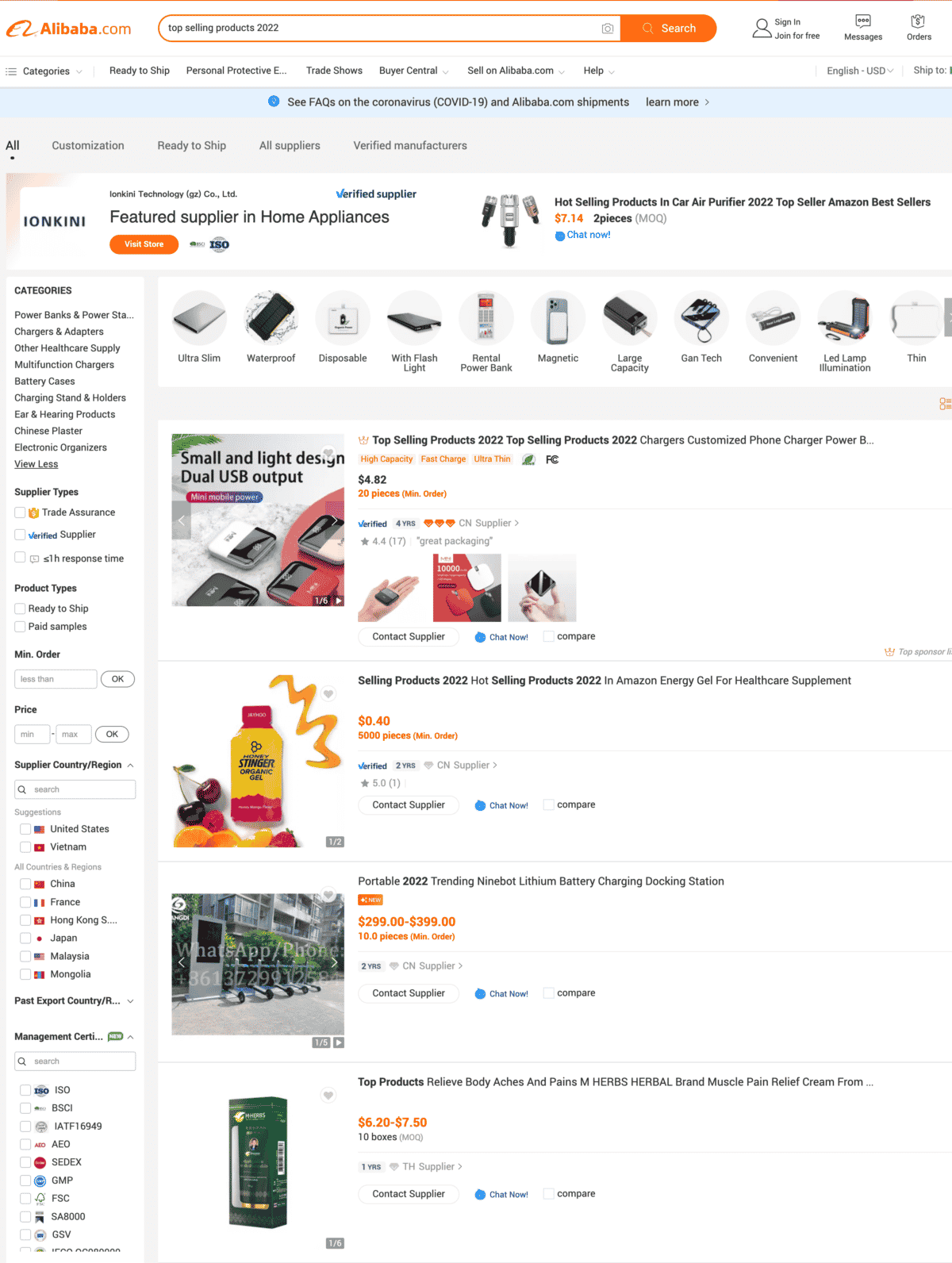This image is a screenshot taken from a computer, displaying the Alibaba.com website in a vertical portrait orientation. The small font size and compact user interface elements indicate that it is viewed on either a laptop or desktop computer rather than a mobile device. 

In the upper left corner, the Alibaba.com logo is prominently featured with bright orange text on a white background, accompanied by the Alibaba mascot face logo. To the right of the logo, a search bar is displayed where the user has input the query "top-selling products of 2022." Adjacent to the search bar is a bright orange search button. Following this, there are additional buttons for account sign-in, messages, and orders.

The main content of the screenshot highlights a banner advertisement for a featured supplier in the Home Appliances category, specifically showcasing "Ionkini." This banner promotes "hot selling products" in the Car Air Purifier segment for 2022, listed as top sellers on Amazon. Below the banner ad, multiple product listings related to the search query are visible, including items such as "Selling Products 2022," "Porto 2022," and "Trending Lithium Battery."

The overall user interface is well-organized, with a clear focus on promoting top-selling and trending products for the year 2022.